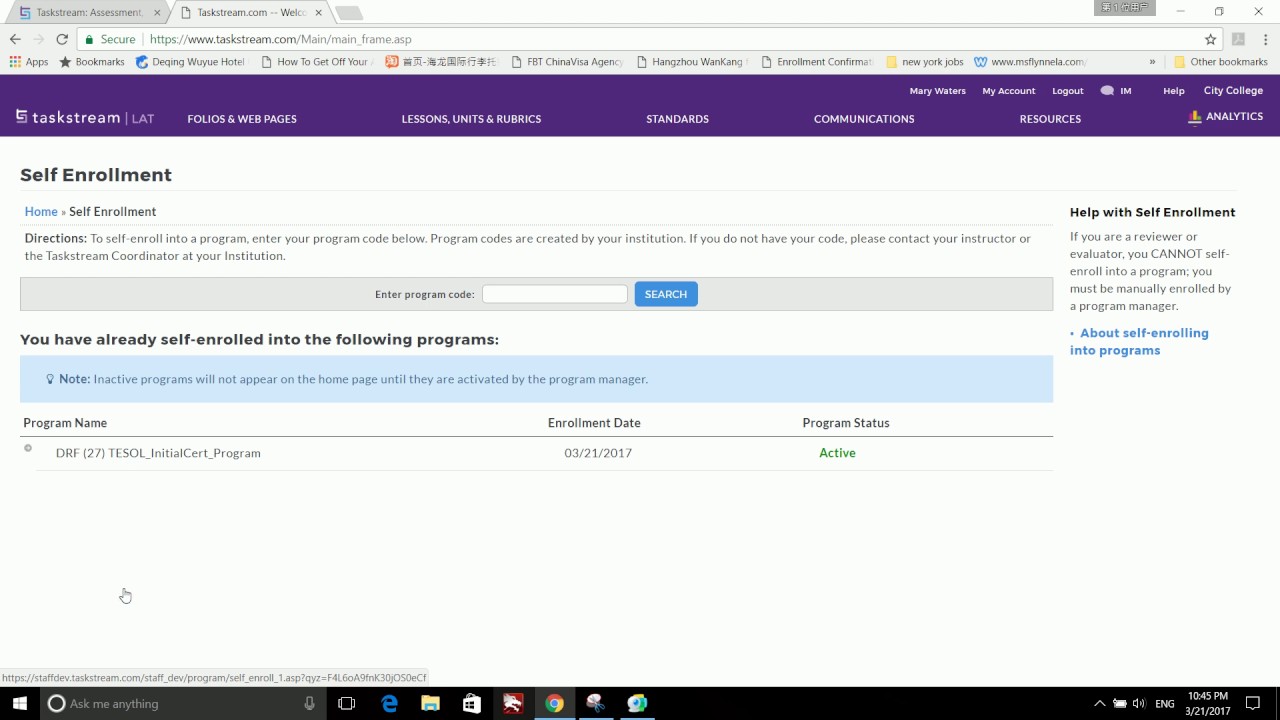The image shows a screenshot of a webpage from TaskStream.com, specifically the self-enrollment page. The top left of the page features a title that reads "Self-Enrollment." The main content area provides directions for users to self-enroll into a program by entering their program code. The text clarifies that program codes are generated by the institution and advises those without a code to contact their instructor or TaskStream coordinator.

Below this instructional text, there is a field where users can input their program code, accompanied by a blue search button. Following this section, the page indicates already self-enrolled programs under a header with a note in a blue box. This note warns that inactive programs will not appear on the homepage until activated by the program manager.

The page lists enrolled programs in a table with three columns: Program Name, Enrollment Date, and Program Status. According to this table, the user is enrolled in the "DRF27 TESOL Initial Cert Program," with an enrollment date of March 21, 2017, and a status of "active."